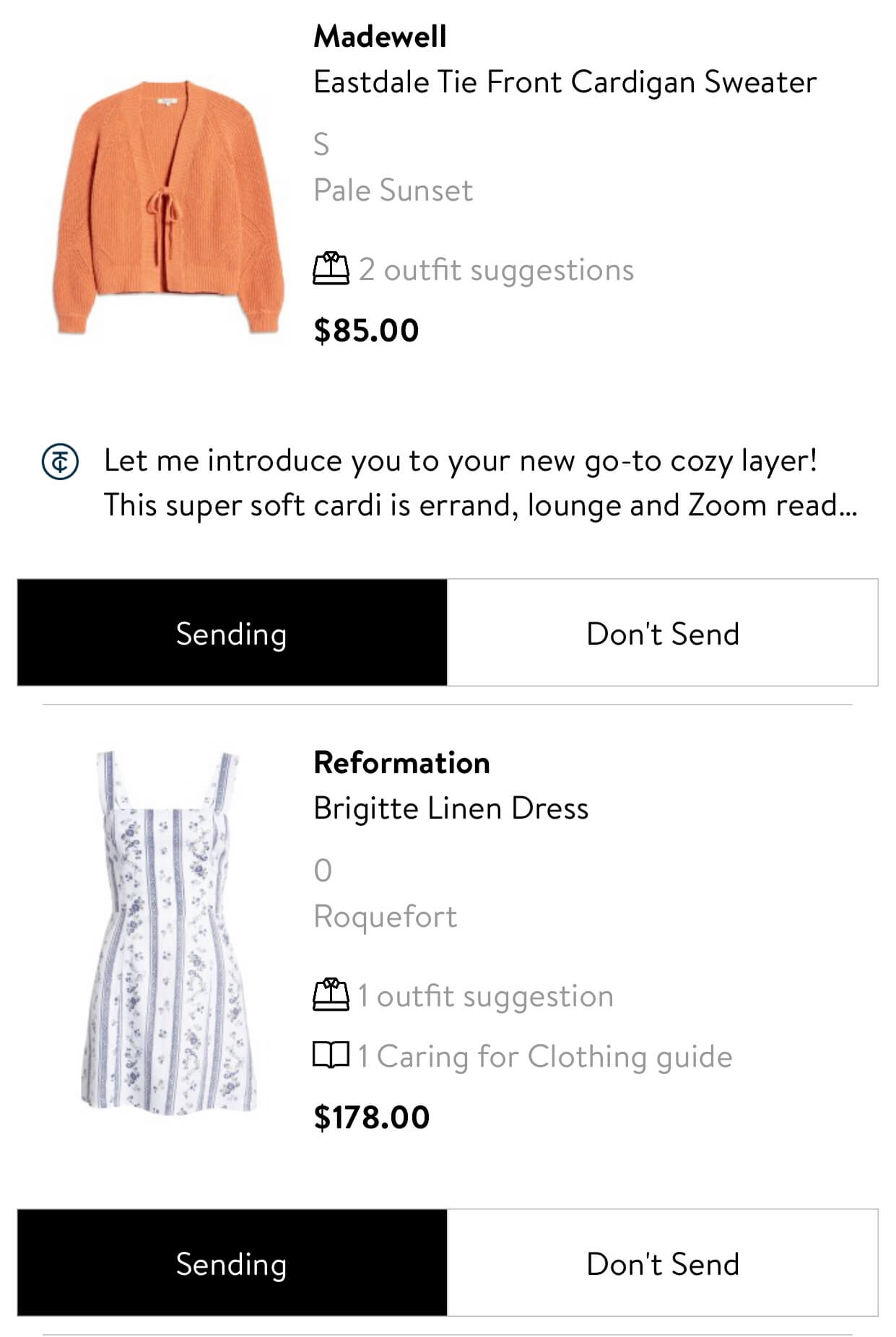The image depicts an online shopping interface with a white background, showcasing two products in the top right corner. The first product, accompanied by a description written in black text, is a "Madewell Tie-Front Cardigan Sweater." The description highlights that it is a super-soft cardigan, perfect for lounging, errands, and Zoom meetings. The sweater is a color called "Pale Sunset," which resembles orange, and is priced at $85. The product image is situated on the top left of the description.

Below the description, there are two interactive buttons: the "Send" button on the left, which is highlighted in white text against a black background, and the "Don't Send" button on the right, written in black text on a white background.

The second product featured is the "Reformation Breccia T-Dress," described in black text. This dress is suitable for various outfits, coming with a clothing care guide. The dress is colored "Rickford," which visually appears as light blue, and is priced at $178. The image of the dress appears on the left side of its description. Similarly to the first product, there are two interactive buttons below the dress description: the "Send" button on the left, in white text on a black background, and the "Don't Send" button on the right, in black text on a white background. The overall design maintains a clean and minimalistic aesthetic with a white background across the image.